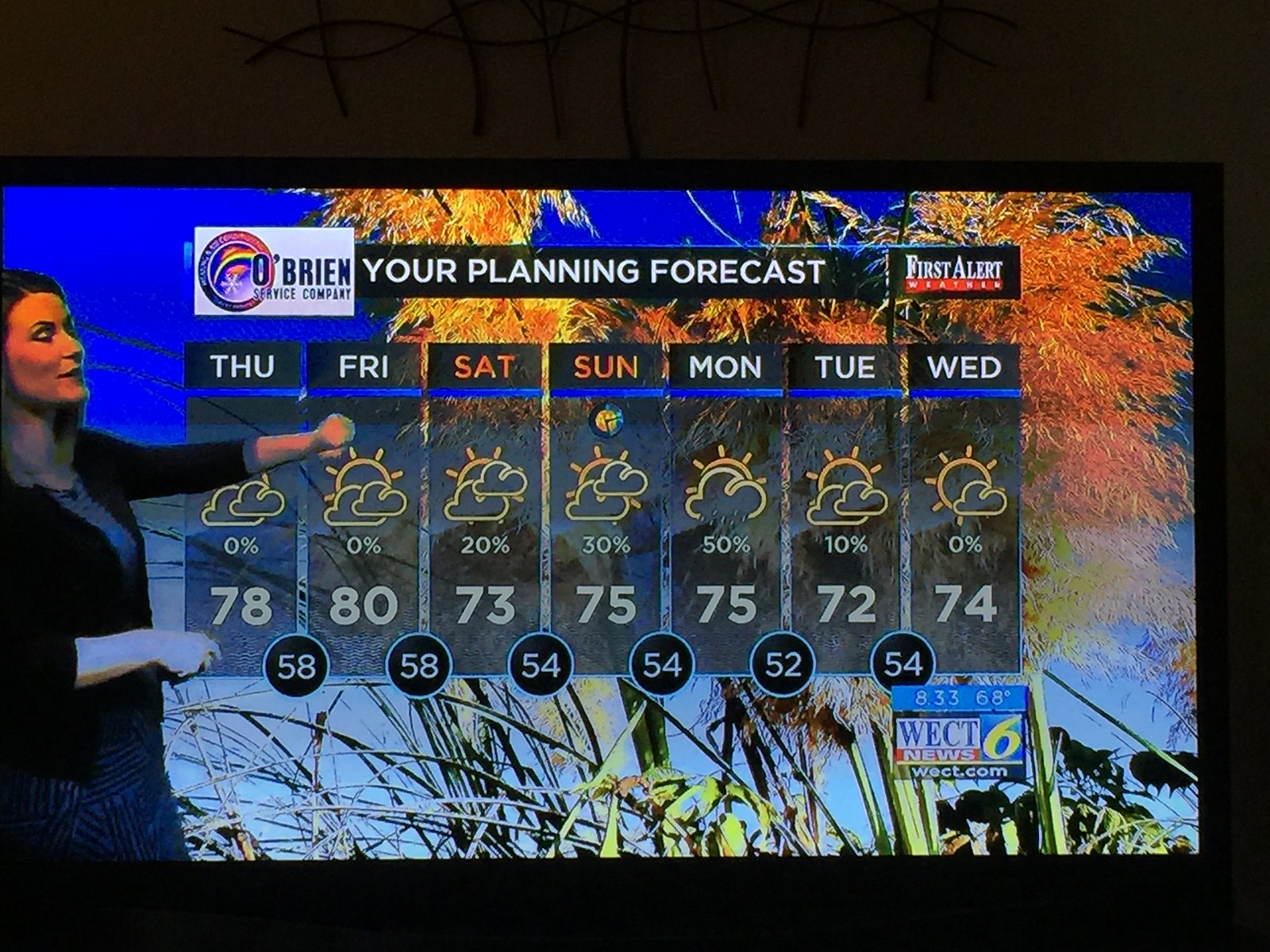The photograph captures a television screen displaying a detailed weather forecast on a flat-screen TV against a white wall. The TV is black, and on its screen, a white woman is delivering the weather report. Positioned on the left side of the screen, she wears a black sweater with mid-forearm sleeves paired with a black and gray striped skirt. The top left corner of the screen features "O'Brien Service Company," and below that, the phrase "Your Planning Forecast" is displayed in white, all-capital, sans serif font. The top right corner reads "First Alert Weather," indicating the nature of the forecast.

Central to the forecast, a seven-day weather outlook is outlined, with each day of the week—Thursday through Wednesday—accompanied by respective temperature highs ranging from 72 to 80 degrees Fahrenheit. Below, the chances of precipitation are noted, varying from 0% to 50%. The weather report includes graphical elements like suns and clouds to visually represent the expected conditions.

In the bottom right corner, the station identifier "WECT News 6" is visible. The background image for the forecast features vibrant imagery of orange foliage, green stems, and large green blades of grass, adding a touch of natural aesthetic to the presentation.